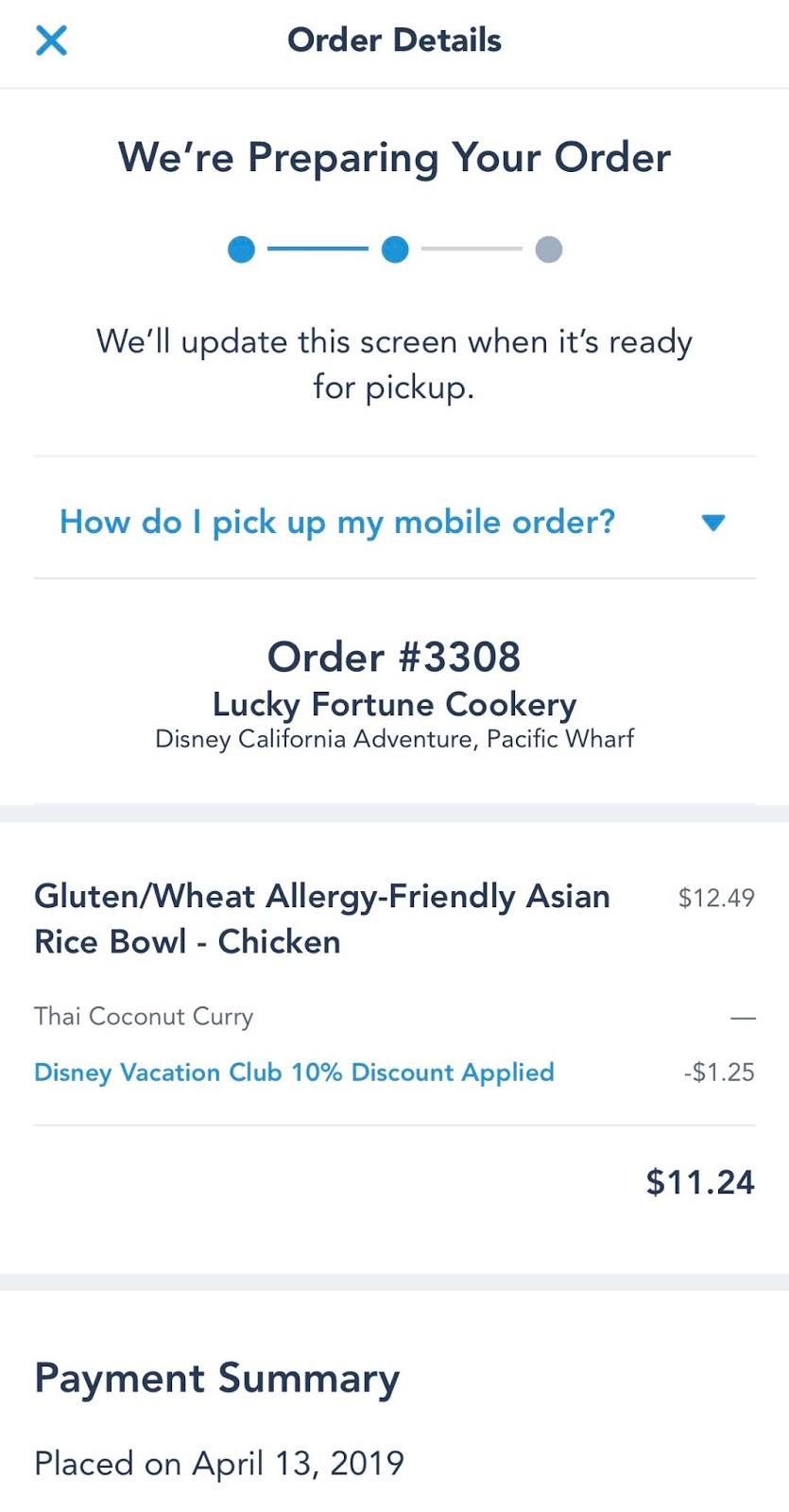Against a clean white background, the image features a detailed order summary for a mobile order. In the top left corner, a blue "X" icon is visible. Directly next to it, in navy blue font, the words "Order Details" are displayed. Below this, a thin gray line spans the width of the image. 

Next, in navy blue, it states "We're preparing your order," followed by a progress bar composed of three circles: the first two are filled in blue with a connecting blue line, while the last circle is gray with an accompanying gray line, indicating the order is not yet complete. 

Beneath the progress bar, further instructions in navy blue state, "We'll update the screen when it's ready for pickup," followed by another thin gray line. The next line in blue reads, "How do I pick up my mobile order?" with a blue rectangular icon pointing downwards.

Another gray line separates this section from the subsequent details, which list the order number "3308" preceded by a pound sign. Underneath, the order name "Lucky Fortune Free" is noted. Below, the location "Disney California Adventure, Pacific Wharf" is specified, bordered by another thin gray line. 

In navy blue, the food item "Gluten/Wheat Allergy-Friendly Asian Rice Bowl – Chicken" is listed with a price of $12.49. Underneath, in black, "Thai Coconut Curry" is mentioned, followed by a discount statement in light blue: "Disney Vacation 10% Discount Applied," subtracting "$1.25" from the total. This section concludes with another thin gray line.

At the bottom of the detailed summary, the total amount is displayed in black as "$11.24." Finally, a gray border separates the payment information, which notes the order was placed on April 13, 2019.